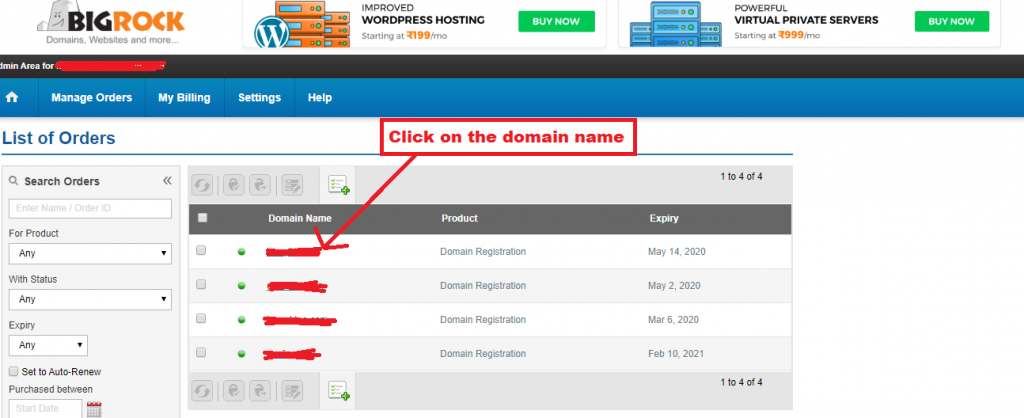The website displayed is for BigRock. At the top of the image is a menu bar where "BigRock" is prominently displayed in capital letters, with "Rock" in orange and "Big" in black. The menu displays options for "Domains," "Websites," and more. To the right side of the menu bar, there is a promotional icon along with text advertising "Improved WordPress Hosting for $1.99 a month," accompanied by a green "Buy Now" button. Next to this, an additional offer for "Virtual Private Servers" is showcased, also featuring a green "Buy Now" button.

Below the menu bar, there's an administrative area with the user's name obscured by a red line. Following the admin section, there's a secondary menu set against a blue background, featuring options including "Home," "Manage Orders," "My Billing," "Settings," and "Help."

In the main content area, a list of orders occupies the majority of the page. This section allows users to search for orders by product, with filters for status and purchase dates. The detailed list includes columns for domain names, which are clickable, along with the associated product and expiration date. A red arrow points to one of the domain names for emphasis. The page being viewed is noted as page 104.